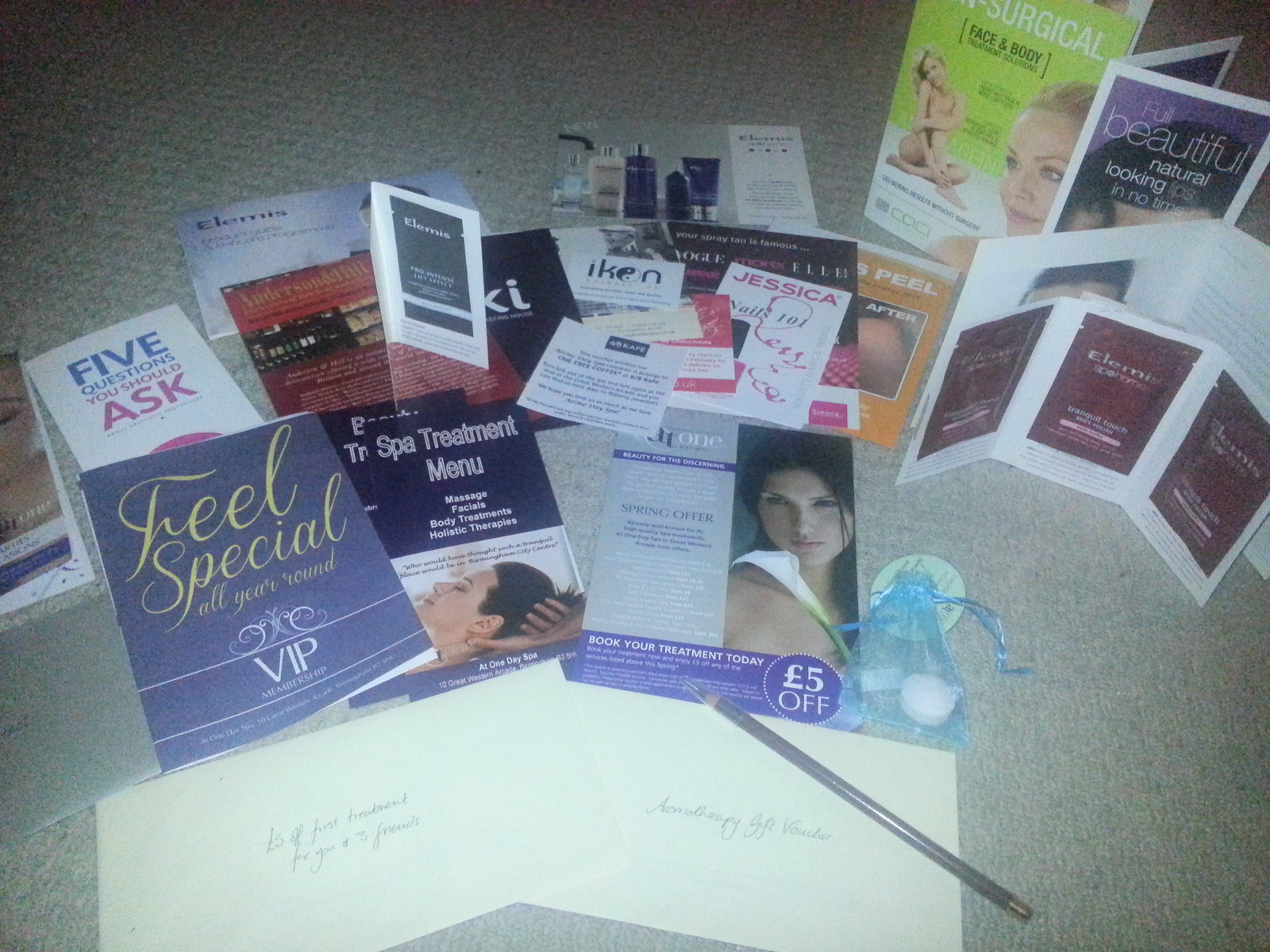The image showcases a gray-patterned table or carpet, arrayed with a variety of colorful brochures and business cards, all centered around beauty and wellness. The diverse flyers display images of makeup, women's faces, and phrases like "beautiful," "natural," and "full beautiful natural looking in no time." Some of the brochures include titles like "Feel Special All Year Round VIP Membership," "Five Questions You Should Ask," and "Spa Treatment Menu" with services such as massages, facials, body treatments, and holistic therapies. Additionally, there is a surgical brochure depicting a nude woman with her knees up against her chest. The scene suggests a display at a convention or exhibition, emphasized by neatly arranged and casually strewn materials, including two white envelopes with an eyeliner pencil on top and a blue bag containing a sample soap or candles.